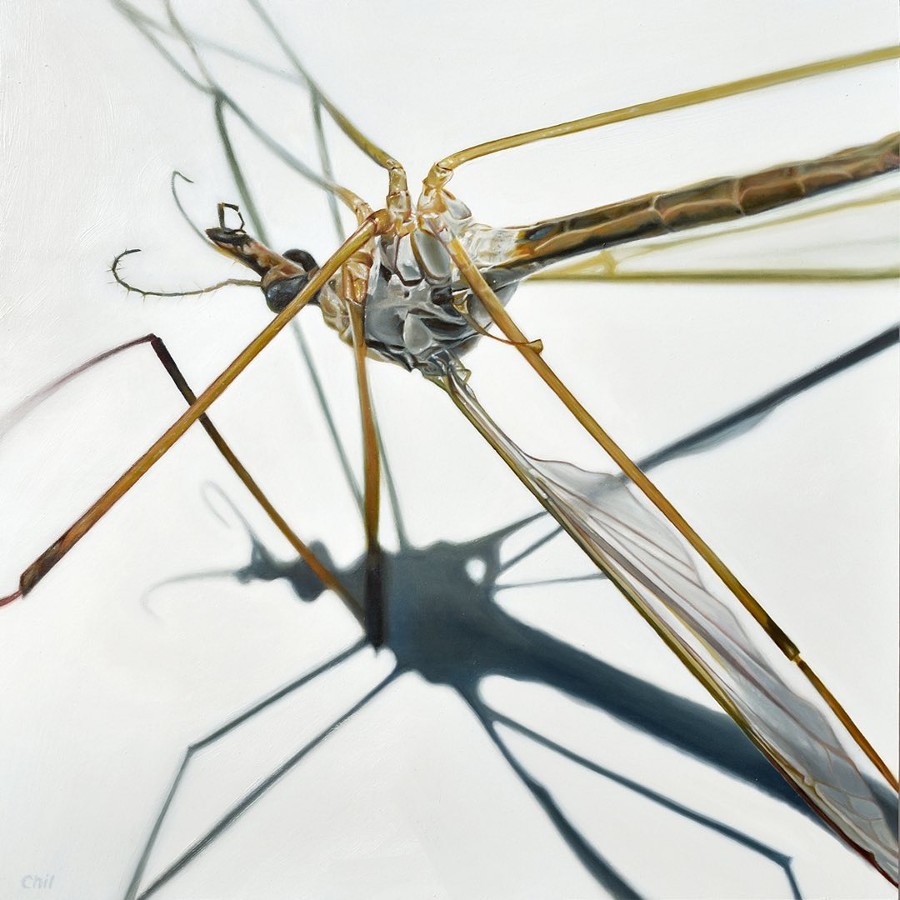The close-up image depicts an insect, likely a mosquito or a similar type of mosquito-like bug, positioned on its back against a stark white background. The white background provides a stark contrast, highlighting the shadow cast by the insect's body below it. The insect's body is predominantly grayish, with translucent qualities that reveal intricate internal structures. Its legs are tan, appearing almost golden against the body, and are notably straw-like in their transparency. 

The insect has a total of six legs, though some descriptions suggest that only four might be clearly visible. It features a long snout with a black tip, which likely serves as its mouth, and two black eyes. Additionally, the insect has a pair of barbed antennae. One of its delicate, transparent wings rests on the ground, while the other appears to be elevated, showing visible veins or structural supports. The abdomen is described as having a mix of black and tan coloration. The absence of any contextual elements aside from the white background and the insect’s shadow enhances the focus on the detailed, albeit somewhat ambiguous, anatomy of the insect.